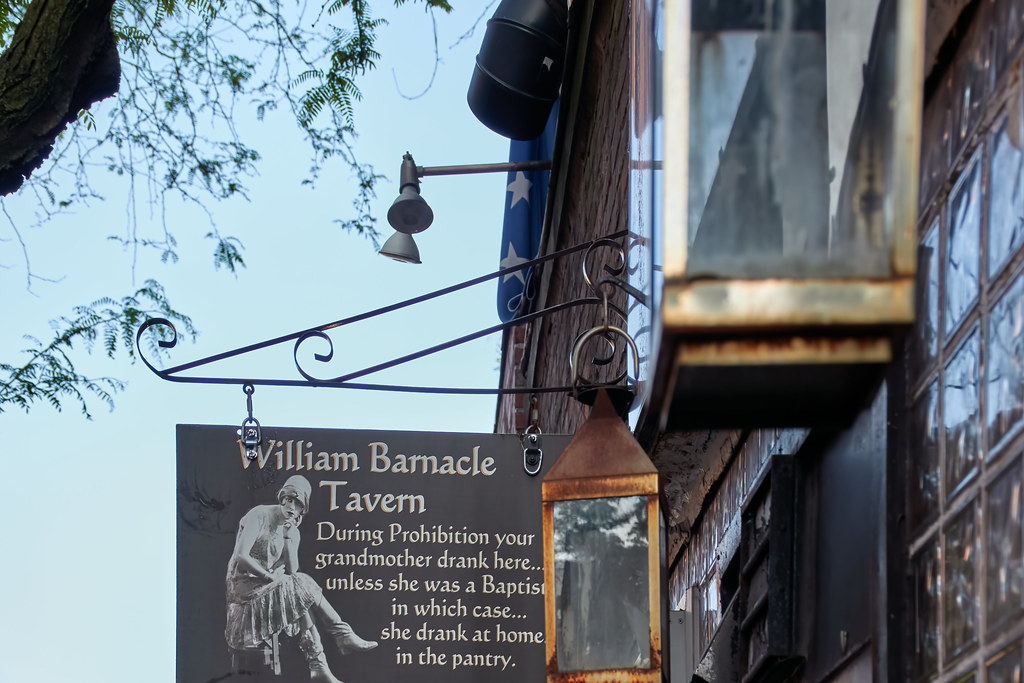This full-color outdoor photograph, taken shortly after dawn or around dusk, depicts the William Barnacle Tavern. The tavern, which is a brown building with thick, heavy windows featuring grids, stands prominently on the right. Adorning the building are a couple of old-fashioned oil lamps and two modern electric lights in the upper part of the frame. Nearby, an American flag and a speaker can be seen. The scene is enhanced by a tree visible in the upper left corner and an overall blue sky indicating a calm evening or early morning setting.

A key feature of the image is an eye-catching sign for the William Barnacle Tavern, showing a depiction of a 1920s flapper girl sitting with her head resting on her hand, legs crossed, and a somewhat melancholic expression. The sign humorously states, "During Prohibition your grandmother drank here. Unless she was a Baptist, in which case she drank at home in the pantry." The sign, predominantly white, stands out against the rustic charm of the tavern's exterior lit by the antique lanterns below it, which are described as rusty brown gold and currently not illuminated.